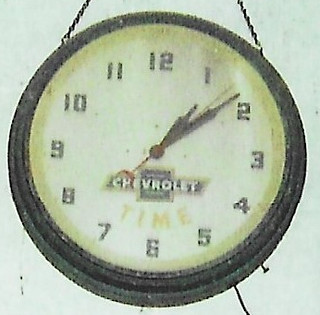A vintage analog wall clock, evocative of those commonly found in schools or businesses, hangs from a chain. The clock features a sleek black exterior and a small black winding cord hanging from the bottom right, allowing for time adjustments. The clock face is white with bold, black numerals and includes black hour, minute, and seconds hands. Uniquely, the second hand is accented with a red center pivot and a red back end. The clock proudly displays the Chevrolet logo in black, accompanied by the word "Chevrolet" in a slightly faded orange-yellow hue below, followed by the word "Time" in the same vintage coloring.